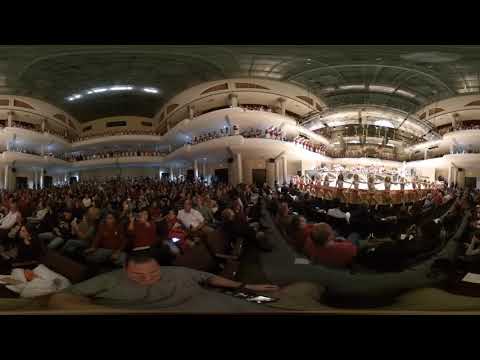This panoramic photo captures the vast interior of a three-level auditorium from the view of the stage. The auditorium, predominantly white with its walls and supporting pylons, features multiple rows of audience members seated on the ground level. Five large sections of seats extend towards the back, evoking the rounded, layered design reminiscent of the Millennium Falcon. The upper two levels are broad, round-shaped balconies filled with spectators. Additional details highlight the green-colored ceiling with metallic elements, contributing to the structural aesthetics. Towards the right side, some women seem engaged in a performance on stage. Dominating the foreground is a heavy-set man in a gray short-sleeved T-shirt, seated closest to the stage, with noticeable black short hair. The scene is lively, as many attendees in red add a burst of color amidst the white interior.